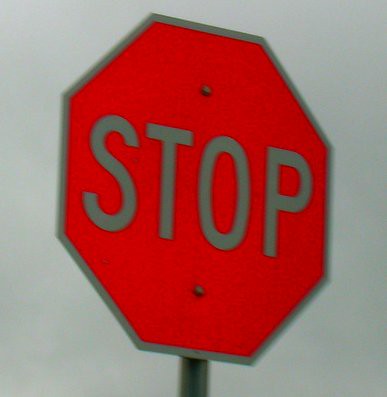This image features a distinctly reflective stop sign, characterized by its intense orange-ish red hue that differs from the more commonly seen darker red signs. The sign is bordered by a pronounced gray rim and displays the word "STOP" in light green letters that match the green border. The background possesses a light grayish tone, offering contrast to the vibrant stop sign, which is slightly angled to the right. Noticeable within the top and bottom centers of the sign are two round rivets securing it to a dark gray pole. The reflective quality of both the sign and its lettering suggests that it is designed to be highly visible, even in low-light conditions.